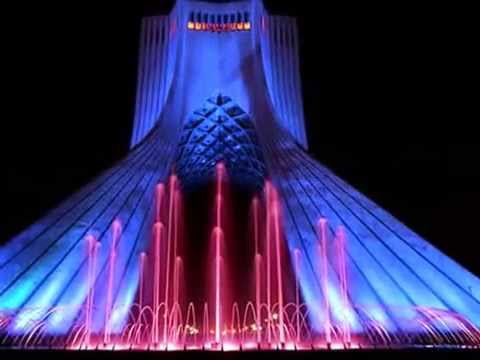The photograph features a striking blue building with a unique, butte-like shape, tapering from a broad base to a narrower top. The structure is adorned with white streaks near the bottom, possibly from light reflections. On the left and right sides, the building appears to have slides. In the middle section, there's an artful pot with a lattice structure, contributing to the artistic aesthetic. Tiny windows dot the upper part of the building, glowing with an orange-yellow hue, possibly hinting at an observation deck. The scene is vividly lit with red and pink lights, and in front of the building, a grand water fountain displays a mesmerizing show. Streams of water shoot upwards, some in graceful arches, enhancing the dynamic and colorful foreground against the deep blue of the evening. The dark area at the base gives an impression of the building standing on two legs with a hollow center, adding to its architectural intrigue.